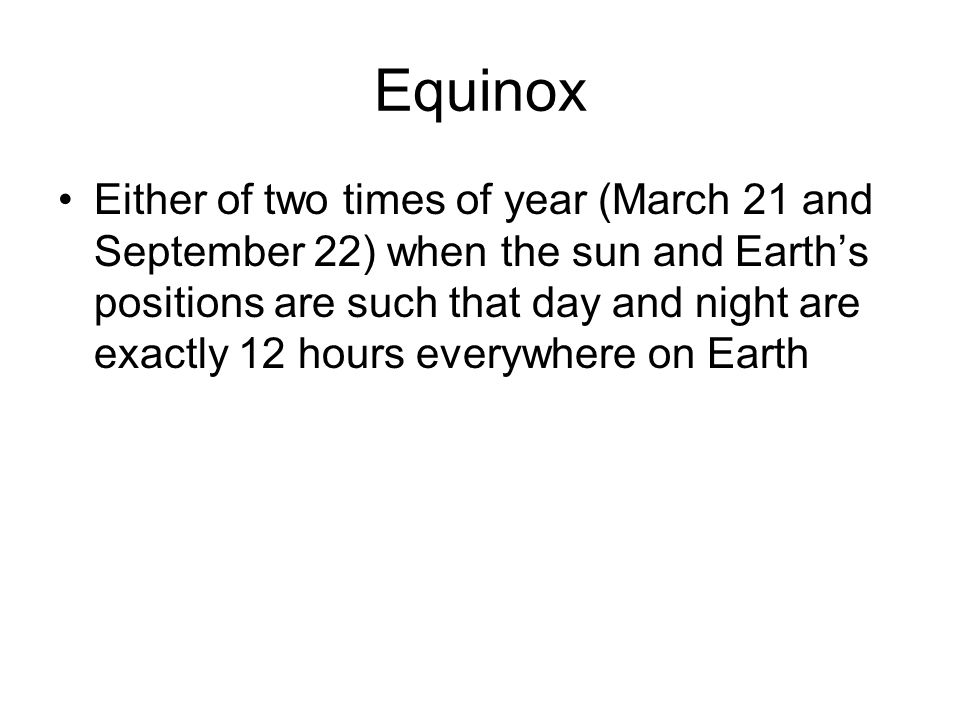The image consists solely of black text on a white background. At the top, in large font, the heading "Equinox" (with a capital "E") is prominently displayed. Beneath it, in a smaller sans-serif Arial font, a single bullet point presents the definition: "either of two times of year, March 21st and September 22nd, when the sun and Earth's positions are such that day and night are exactly 12 hours everywhere on Earth" (the capital 'E' is used for each instance of the word earth). Besides the parentheses around the dates, there is no other punctuation. There are no images, borders, frames, or special effects accompanying the text.